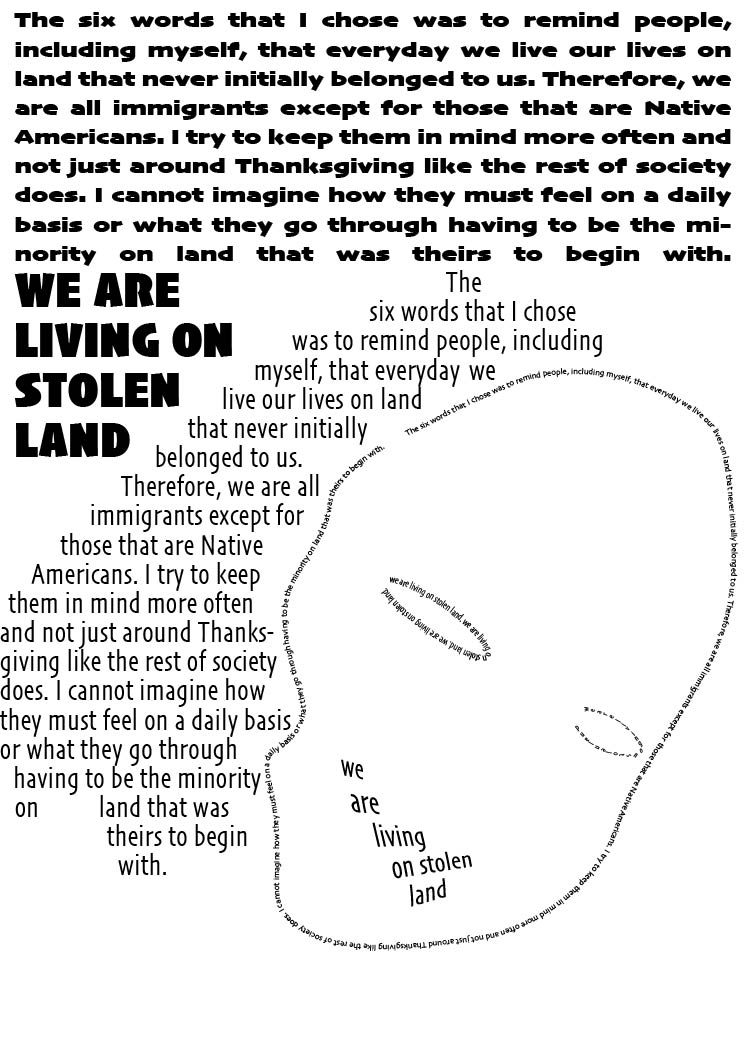The image is a portrait-oriented rectangle with a pale, light blue background. At the top, in bold black print, it reads: "The six words that I chose was to remind people, including myself, that every day we live our lives on land that never initially belonged to us. Therefore, we are all immigrants, except for those that are Native Americans. I try to keep them in mind more often, not just around Thanksgiving like the rest of society does. I cannot imagine how they must feel on a daily basis, or what they go through having to be the minority on land that was theirs to begin with." Below this, also in bold black print, the phrase "We are living on stolen land" is prominently displayed on the left. To the right, there is an artistic depiction of a face, formed by the repeated text "The six words that I chose was to remind people, including myself, that every day we live our lives on land that never initially belonged to us. Therefore, we are all immigrants, except for those that are Native Americans. I try to keep this in mind more often, and not just around Thanksgiving like the rest of society does. I cannot imagine how they must feel on a daily basis, or what goes through their having to be the minority on land that was theirs to begin with." The hair of the figure cascades from the top right to the bottom left, with the mouth highlighted by the text "We are living on stolen land." The image lacks specific facial details but contains the outlines of eyes and a mouth created through the text, emphasizing the message of living on lands that were originally Native American territories.